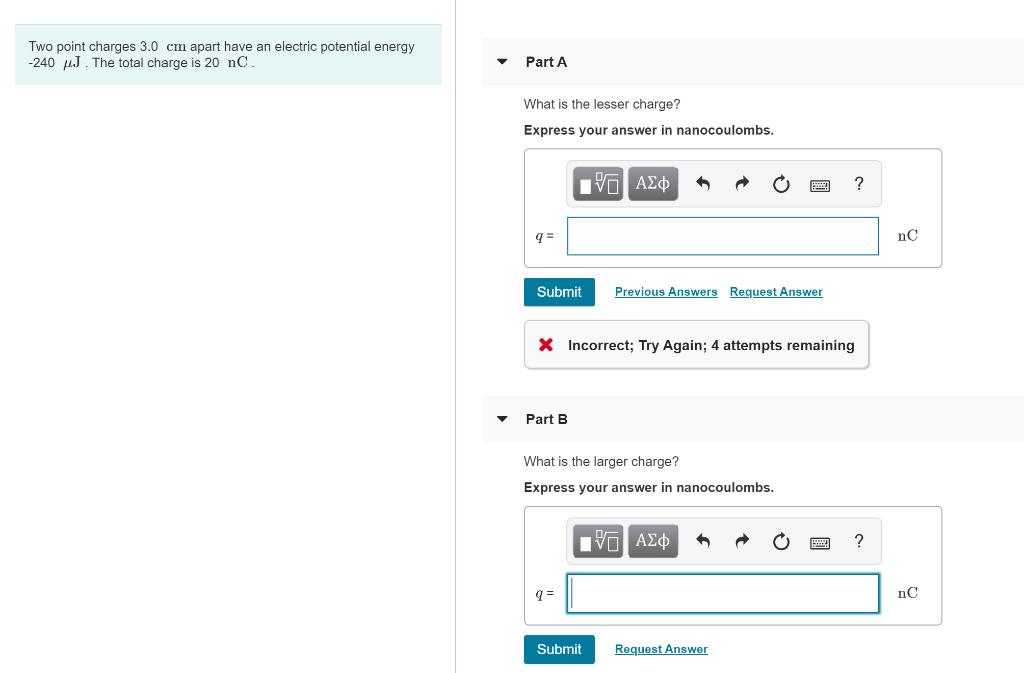The image is a portion of a highly technical screenshot that appears to be related to a physics or electrical engineering problem. The layout is divided into two sections by a thin vertical line.

**Left Section:**
- At the top, there is a light blue rectangle.
- Inside the rectangle, in gray font, it reads: "Two point charges, 3.0 cm apart, have an electric potential energy," followed by a mathematical equation.
- Below, it states: "The total charge is 20N, C," indicating 20 nanoCoulombs (Nₑ C).
- The rest of the left section remains blank.

**Right Section:**
- At the top, there is a very light gray rectangle.
- On the left side of this rectangle, it says "Part A" in black font.
- To the left of "Part A," there is an inverted triangle, signifying a dropdown menu.
- Beneath this is the question: "What is the lesser charge?" followed by the instruction to "Express your answer in nanoCoulombs (nAᴘCᴏᴜʟᴏᴍʙs)."
- Below the question is a rectangle containing various mathematical equations and symbols.
- There is a blue rectangle with the word "Submit" in white.
- Below "Submit," two hyperlinks appear in blue font and are underlined: "Previous Answers" and "Request Answer."
- Underneath these, in a gray rectangle, there's a red 'X' sign next to the text "Incorrect, try again. Four attempts remaining."
- Further down is "Part B," which follows a similar format:
  - The question: "What is the larger charge?"
  - An instruction to "Express your answer in nanoCoulombs (nAᴘCᴏᴜʟᴏᴍʙs)."
  - A similar arrangement of a text box for equations and a "Submit" button.

The overall format indicates an interactive problem-solving environment typical for educational or instructional software.